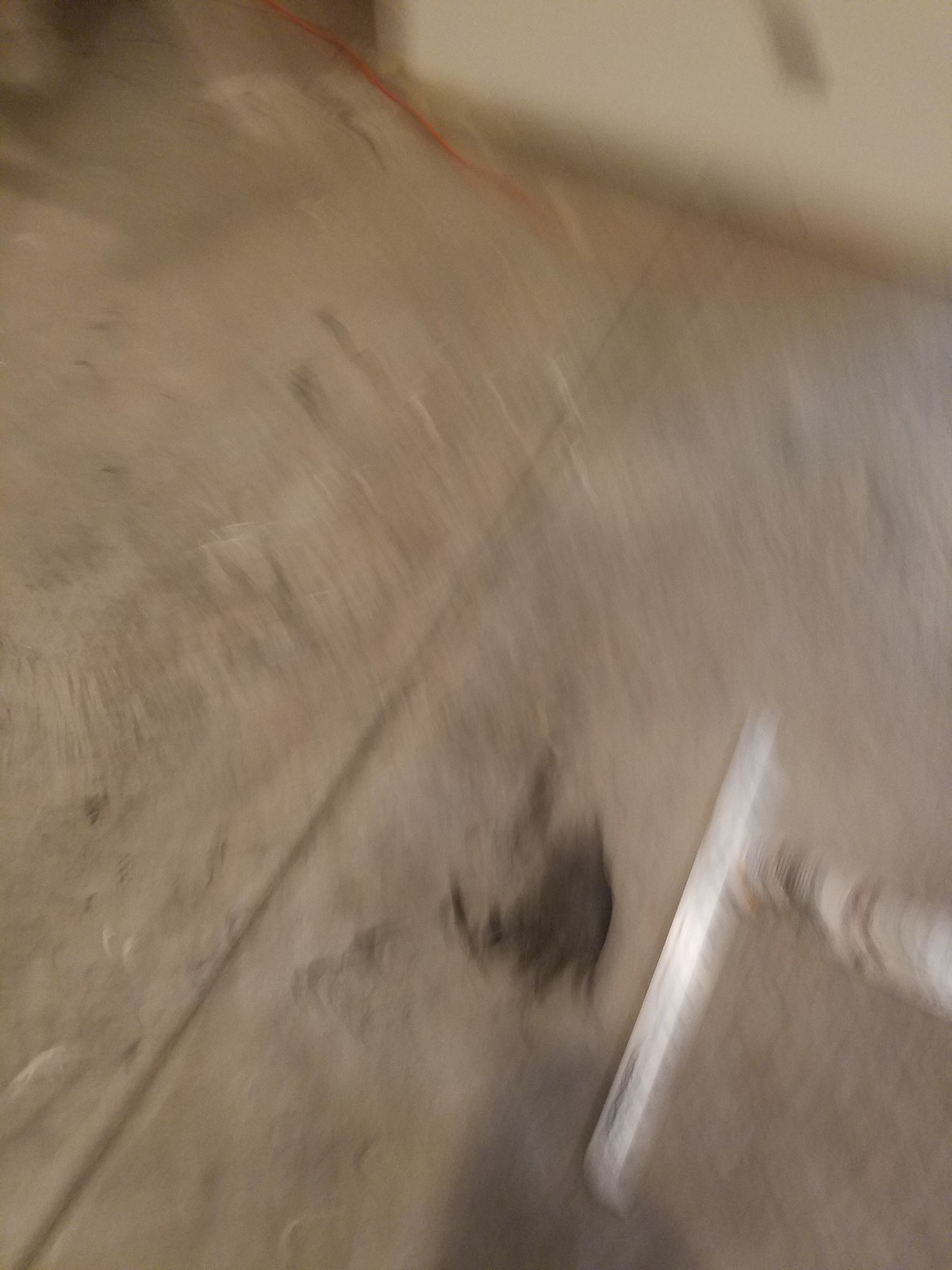This photograph, although blurry, predominantly features a range of light brown to gray hues, suggesting it was taken of the ground. The image appears to capture a section of a sidewalk, identifiable by a discernible expansion joint. Near this joint, there is an area covered with some sort of dark brown material, though its exact nature is obscured by the blurriness. Adjacent to this dark brown material lies an indistinct white or silver object, potentially the nozzle of a vacuum cleaner, but its precise form and function are difficult to ascertain due to the lack of clarity.